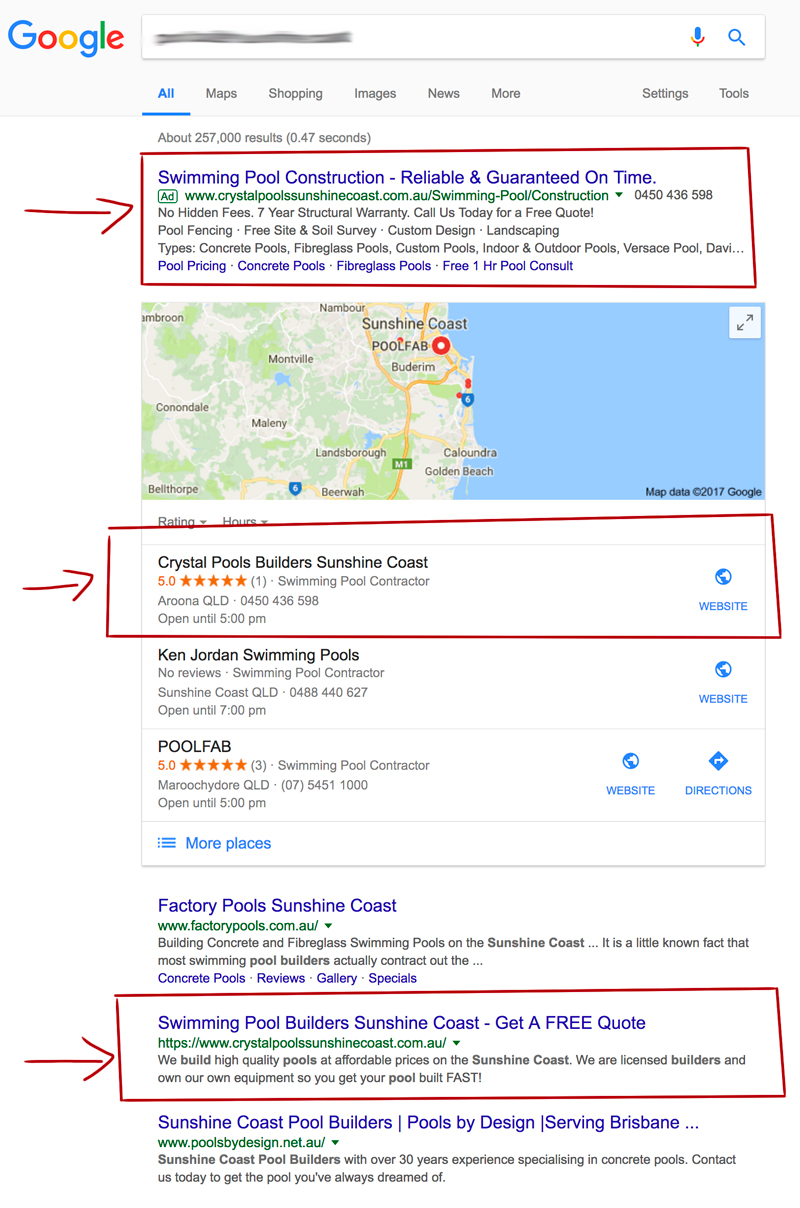**Detailed Caption:**

This image is a screenshot of a Google search results page. The text entered in the search bar is blacked out, but the standard Google logo appears prominently at the top, with its familiar red, yellow, blue, and green letters. Below the search bar, the entire top section is highlighted in blue, and the usual navigation options—Maps, Shopping, Images, News, More, Settings, and Tools—are displayed.

The search yielded approximately 257,000 results in 0.47 seconds. A red arrow is pointing to the top result, which is an advertisement, outlined with a red box. The ad reads "Swimming Pool Construction - Reliable and Guaranteed on Time" with the word "Ad" in green next to it. The ad's URL is www.crystalpoolsunshinecoast.com.au.eu and includes a contact number (0450-436-598). The ad emphasizes "No hidden fees," a "Seven-year structural warranty," and offers a "Free quote" along with various services such as pool fencing, site and soil surveys, custom designs, and landscaping. It also lists types of pools they build: concrete, fiberglass, custom, indoor, outdoor, and specific types like "Versace pool" and "Devi."

A map appears below this ad, highlighting the Sunshine Coast area with various locations marked including Buderim, Nambour, Landsborough, Caloundra, Golden Beach, Montville, and Beewah. Pool Fab is prominently marked in capital letters. The bottom of the map indicates it uses data from 2017 Google.

Another section enclosed by a red box, pointed out by a red arrow, highlights "Crystal Pools Builders, Sunshine Coast" with a 5.0-star rating from one review, listed as a swimming pool contractor in AR Aruna QLD. It provides the same contact number (0450-436-598) and notes operating hours until 5 p.m. A website link is provided.

Directly below, the listing for "Ken Jordan Swimming Pools" mentions there are no reviews. This contractor is located on Sunshine Coast, QLD, with a contact number (0488-440-627) and is open until 7 p.m., with a website link available.

"Pool Fab" is another highlighted contractor, boasting a 5-star rating from three reviews, situated in Maroochydore QLD, and can be contacted at (0754-511000). Their operations also end at 5 p.m.

The page continues with a hamburger menu listing further sections. "Factory Pools, Sunshine Coast" is another listing, linking to www.factorypools.com.au and describing their expertise in building concrete and fiberglass swimming pools.

One more red arrow points to a red box surrounding another ad for "Swimming Pool Builders, Sunshine Coast," offering competitive rates, fast building times, and a licensed, well-equipped team.

Lastly, the caption mentions "Signature Sunshine Coast Pool Builders" and "Pools by design," referencing their specialty in concrete pools with over 30 years of experience, listed on www.poolsbydesign.net.au